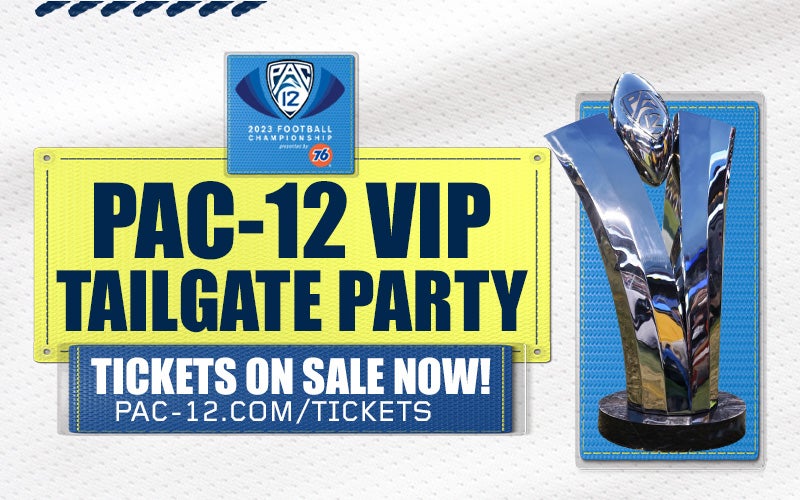This rectangular advertisement features a textured white background resembling athletic jersey fabric with pin-dot holes. At the top-center is a small blue square that reads "Pac-12" with "2023 Football Championship" in white text beneath it. This section includes a small orange circle with the blue number "76," indicating sponsorship. Below the square, a large yellow rectangle with black text announces the "Pac-12 VIP Tailgate Party." Underneath, a thinner blue rectangle with yellow stitching and white text directs viewers to "tickets on sale now" at "pac12.com/tickets." To the right side of the advertisement, there is a tall blue rectangle with white stitching, displaying a silver trophy. The trophy has a black circular base and features an engraved football at the top, with "Pac-12" inscribed on it.